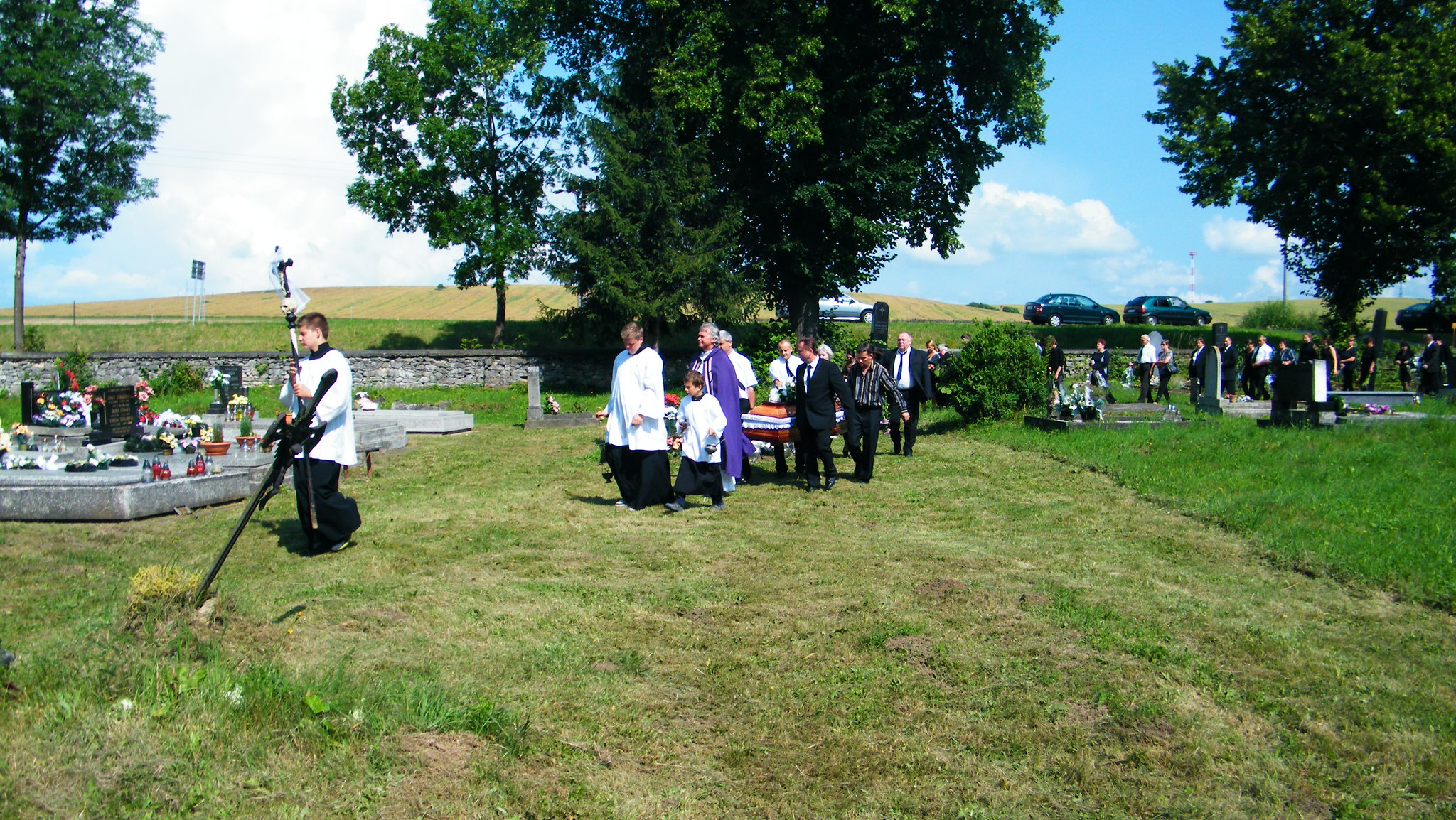In this detailed image set during a funeral procession, we see a central group of people walking towards the camera, solemnly carrying a brown casket. The setting is a large, grassy field, which is sparse in the center but more densely covered towards the sides. Surrounding the mourners are numerous tombstones and headstones, adorned with flowers, candles, and other decorations, particularly noticeable on the left-hand side. The participants include men in black suits with white shirts, some in white robes with black gowns underneath, and a priest wearing a distinctive purple vestment. Additionally, altar boys are present in the procession. In the background, there are various farms and fields, a line of green hills, and a multitude of trees in the middle top of the image and the corners. To the right, two black cars are parked in a line. Above, the bright blue sky is dotted with puffy white clouds. The image captures the serene and somber ambiance of the outdoor funeral, held under daylight. The colors in the scene range from light blue, white, and gray to different shades of green, alongside touches of red, pink, yellow, and purple from the surrounding elements.